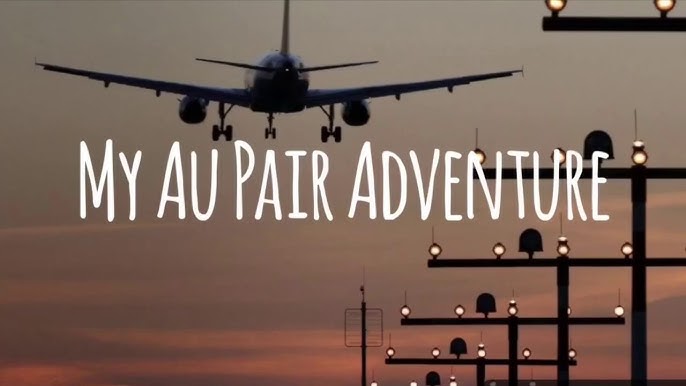The full-color photograph captures a stunning outdoor scene at either dawn or dusk, featuring the dramatic ascent of a commercial passenger plane into a sky ablaze with shades of red and purple. The horizontally rectangular image is unbounded, set against a backdrop solely of sky. Precise lighting elements highlight the scene—both natural light from the low sun and artificial light from black poles topped with illuminated lamps that stretch diagonally from the lower left to the upper right corner. Dominating the center of the composition, bold white text reads "My Au Pair Adventure," hinting at a narrative of international travel for a nanny role. The background sky transitions from a tannish-gray at the top to the vivid reds and purples, adding depth and drama. The plane itself, with blue and white markings and visible black wheels, appears to be soaring away from the viewer, emphasizing the theme of journey and adventure.